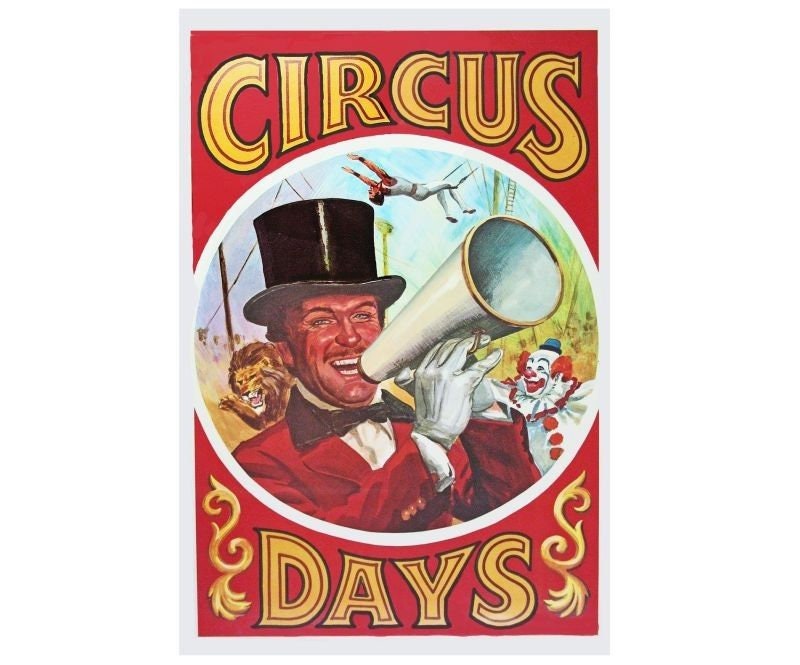The poster is a vintage-styled circus advert with bold colors and a detailed illustration. The central illustration, set within a circular white disc, is positioned against a vibrant red background with a light gray border. The top of the poster reads "Circus" and the bottom "Days," both in an old-fashioned, bubbly yellow font with gold flourishes flanking the word "Days."

The focal point of the illustration is a lively ringmaster stationed on the left side of the circle. He boasts a reddish complexion, a shiny black top hat, a red suit jacket, a white shirt with a dark black collar, a large black bow tie, and white gloves. His brown mustache and white teeth are visible as he exuberantly announces into a white megaphone trimmed with a gold band.

Completing the circus scene, a playful clown stands to the right, dressed in a white gown adorned with red pom-poms and a flouncy collar, and sporting a blue hat and red hair. Above the ringmaster, a trapeze artist performs mid-air acrobatics, while a roaring lion, raising its paw, adds to the spectacle from the left.